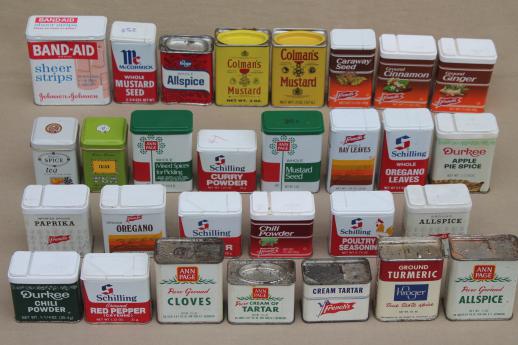This image depicts a meticulously organized collection of 31 metal tins arranged in four neat rows on a light tan surface, likely a table. The collection predominantly consists of various herbs and spices, with a few outliers such as tea canisters and a tin of Band-Aid sheer strips. 

Starting from the back row in the upper left, there is a canister of Band-Aid brand sheer strip bandages by Johnson & Johnson. Moving to the right, the row includes spices like McCormick mustard seed, an unidentified small tin of allspice, two Coleman's mustard tins of varying yellow shades, and concluding with three similarly branded tins that appear to be cardamom seeds, cinnamon, and ginger. 

The third row features a diverse collection including two tins of oriental tea, an Anne Page mustard seed with a green top, a Shilling curry powder, a tall Shilling oregano leaves, and Anne Page bay leaves, and a Durkee's apple pie spice.

The second row presents more spices such as French's paprika, French's oregano, an obscured Shilling spice, an unidentified chili powder, Shilling poultry seasoning, and French's allspice.

The front row, closest to the viewer, displays a lineup of spices including Durkee's chili powder, Shilling red pepper, Anne Page pure ground cloves, Anne Page cream of tartar, French's cream of tartar, a tin of turmeric, and Anne Page pure ground allspice.

The overall arrangement gives a visual inventory of someone's kitchen shelf, laid out in a regimented formation, showcasing the variety and brands of the spices and other items they possess.